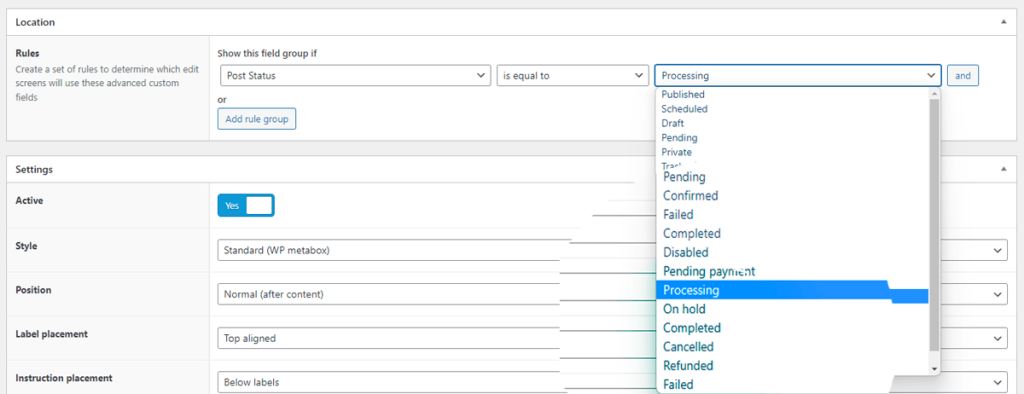The screenshot features a user interface with a gray background. At the top of the image is a long drop-down box, labeled "Location" on the left side in bold black text. To the right of this label is a downward-pointing arrow.

Beneath the drop-down box, there is a gray square. In the top-left corner of the square, the word "Rules" is displayed, accompanied by three lines of small black print. Towards the right side of the gray square, there is a long white rectangle. At the top of this rectangle, in black text, is the phrase "Show the field group if," followed by three horizontally aligned drop-down boxes. At the end of these drop-down boxes, there is a blue button labeled "And." 

To the left of this white rectangle, the word "Or" is displayed, and below it, an "Add full group" button is visible. The third drop-down box in the sequence has been clicked, revealing the term "Processing" and an open drop-down menu that extends over the right side of the screen.

Below this, another white rectangle is present. It is labeled "Settings" in the upper left-hand corner, with an arrow on the right side. Underneath the "Settings" title, there is a list of options on the left, including "Active Style," "Position," "Label Placement," and "Instruction Placement." Corresponding to each option on the right are additional drop-down boxes.